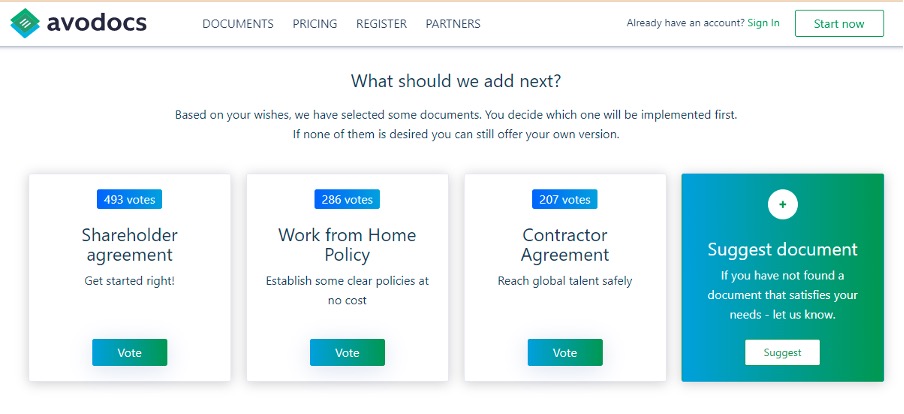Displayed in the image is a website interface for a company named AfroDocs. The top-left corner prominently features the AfroDocs logo and company name. Adjacent to this, in the upper navigation bar, there are several links labeled: "Documents," "Pricing," "Register," "Partners," and an option for existing users to "Sign In." A prominent call-to-action button labeled "Start Now" is located nearby.

Further down the page, there is an interactive section inviting users to contribute to the development of new documents. This section opens with the question, "What should we add next?" followed by explanatory text: "Based on your wishes, we have selected some documents. You decide which one will be implemented first. If none of them is desired, you can still offer your own version."

Below this text, a list of proposed documents is displayed along with their current vote counts:
- "Shareholder Agreement" with 493 votes, accompanied by a "Get Started" button.
- "Work from Home Policy" with 286 votes.
- "Contractor Agreement" with 207 votes.

Users are further encouraged to suggest additional documents if their needs are not met by the listed options, with a button labeled "Suggest." The overall design uses a balanced color palette with shades of white, green, and blue, giving it a professional and approachable appearance.